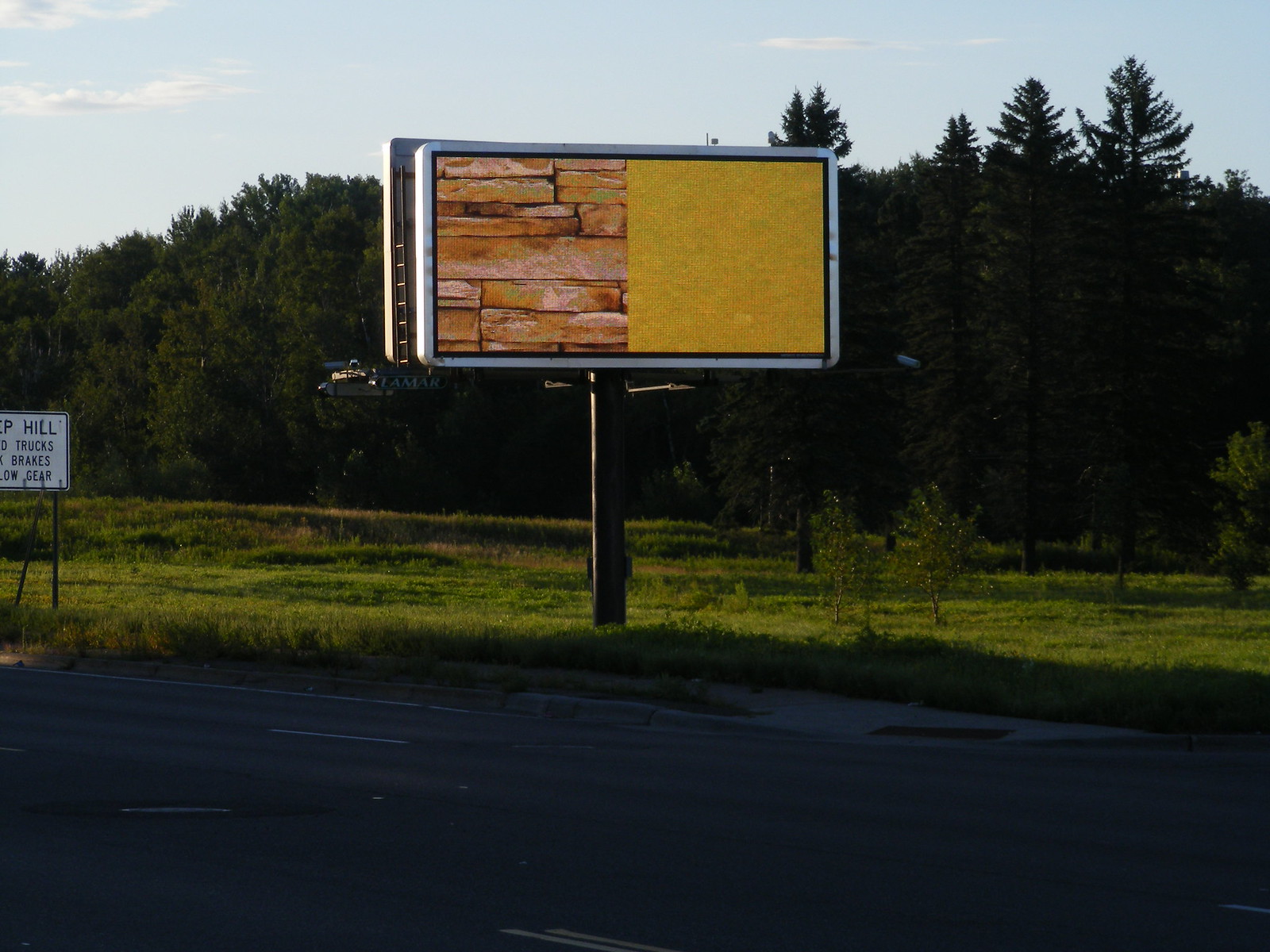The photograph captures a roadside scene during a clear day. The road, made of grey cement, features white painted lines and is bordered by a strip of green, sunlit grass populated with tiny new shrubs. Mature evergreen and leafy trees stand tall in the background. The central focus is a rectangular billboard, mounted on a large black post, divided into two distinct halves: the left side showcases a cobblestone-like brick design in shades of brown, and the right side is a solid, gold-yellow color with a textured appearance. At the base of the billboard, which has a ladder leaning against it, is the word "LAMAR" in green lettering. A smaller, white sign nearby advises "heel trucks brakes and low gear" in black letters. The scene is under a bright blue sky, devoid of clouds, emphasizing the tranquil yet vivid outdoor setting.